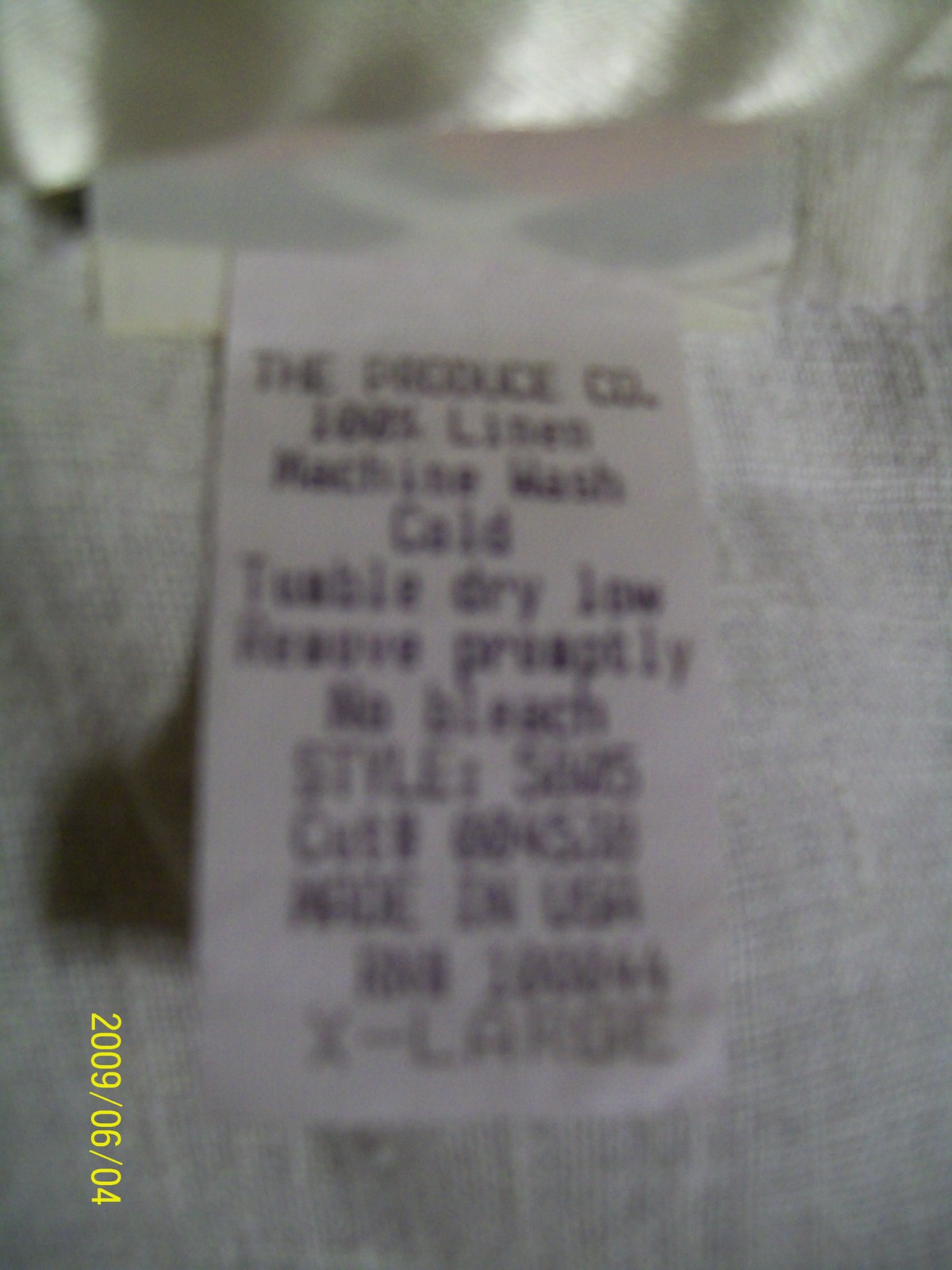This color photograph captures a close-up view of a laundry tag attached to what appears to be a light gray or grayish-white woven fabric, likely a piece of clothing. The central focus is the white garment tag, which is slightly blurry due to zooming. The top of the tag reads "The Produce Company," and it provides care instructions: "100% Linen, Machine Wash Cold, Tumble Dry Low, Reverse Promptly, No Bleach." The rest of the tag's text is partially blurred, but it clearly indicates the size "X-Large" at the bottom in black text. On the bottom left corner of the image, turned sideways, there is a bright yellow date stamp reading "2009/06/04."